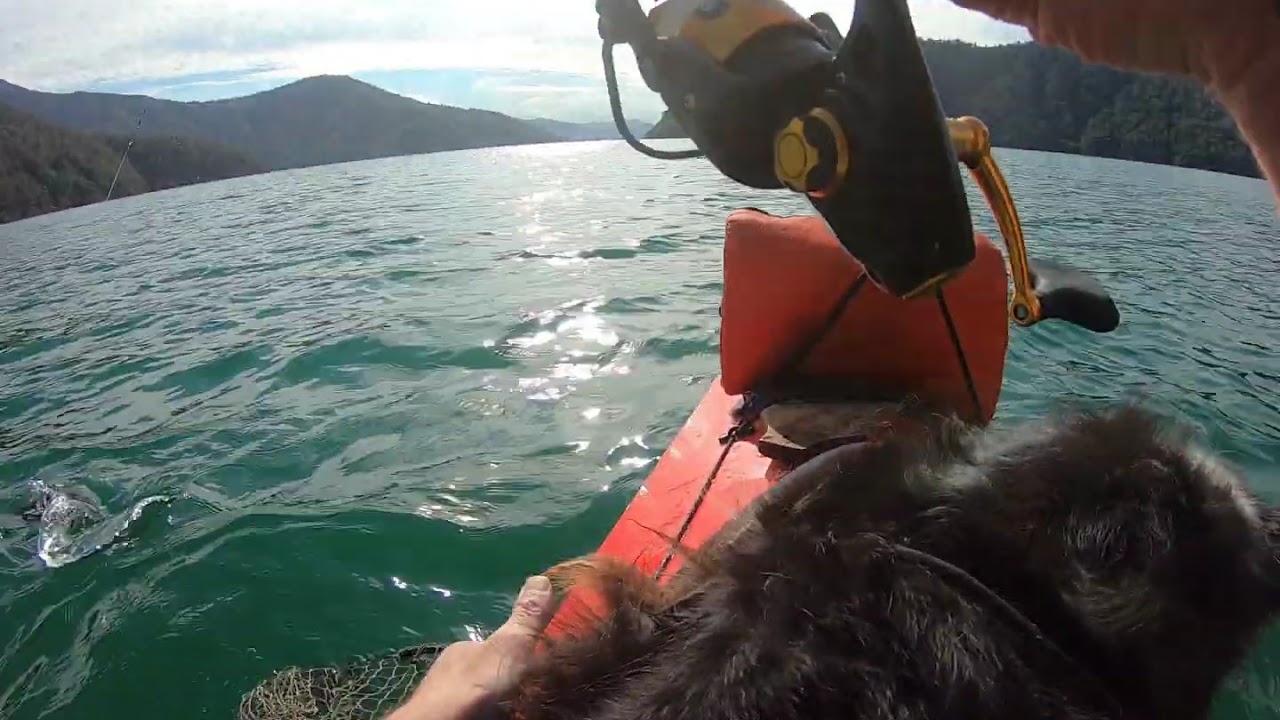In this photograph, taken from the point of view of someone on a boat, a person is fishing in a large, calm body of water, which could be a lake, ocean, or tributary. The person is holding a fishing pole in their right hand and an orange flotation device in their left hand, appearing to be actively reeling in a fish. Sitting on the person's lap or near them is a dog or some kind of furry animal. The scene is captured during daytime under an overcast but bright sky, with sunlight reflecting off the greenish water. In the background, majestic mountains or hills frame the horizon, adding to the serene and picturesque quality of the image. The boat, painted red or orange, includes ropes and controls, and there are no other boats visible in the scene. The overall setting is peaceful and inviting, combining the tranquility of nature with the anticipation of a fisherman’s catch.